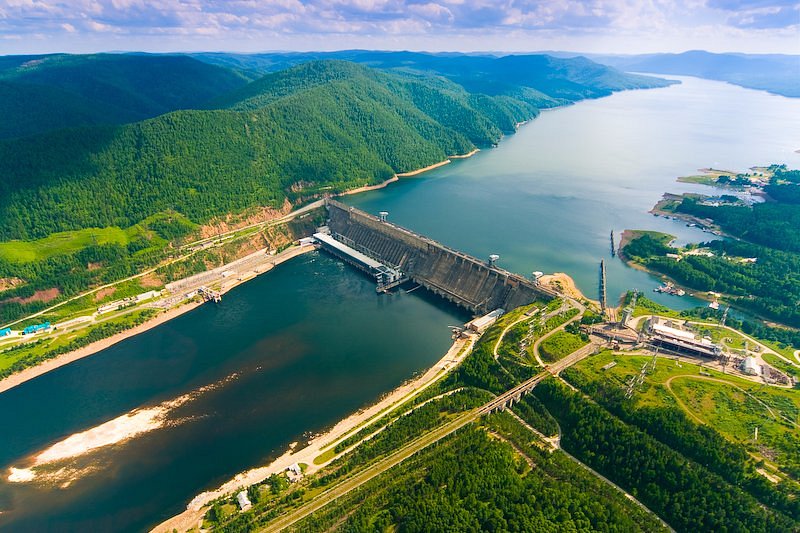The aerial photograph captures a vast, lush mountain range covered in verdant green foliage on either side of a significant body of water. Central to the image is a prominent dam-like structure with water flowing on both sides. In the middle of the water, just left of the dam, lies a sandbar or a section of lighter, possibly foamy water. To the right of the dam, there's a substantial structure, likely a warehouse or a manufacturing facility, with a road leading directly to it. This area also features a small driveway or walkway and several inlets housing tiny buildings and boats. The mountains and surrounding landscape are breathtakingly beautiful, complemented by the vivid green of the trees and the deep blue of the water, punctuated with tan and white patches. Additionally, there are bridges across the water amidst the lush greenery, connecting various parts of the scene. The sky above is dotted with clouds, adding to the overall picturesque quality of the photograph.